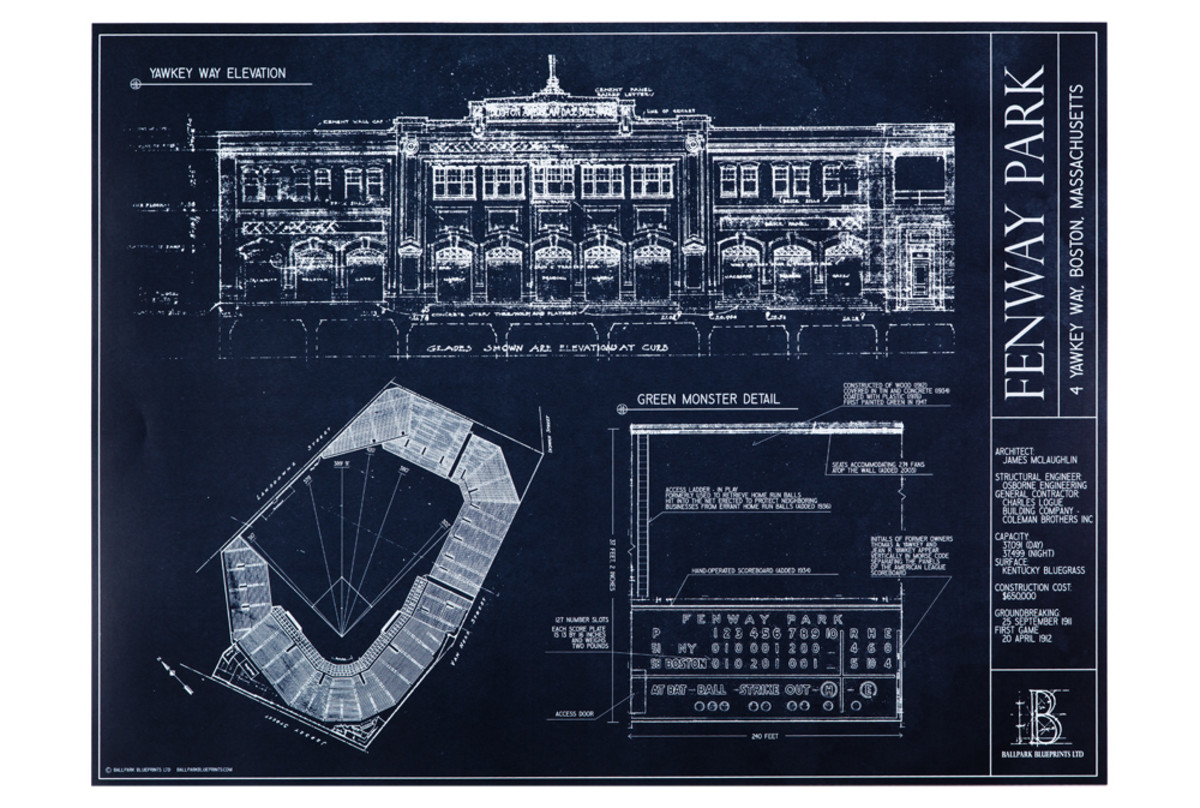The image displays detailed architectural plans for Fenway Park in a rectangular format with a dark navy, almost black background, and white fonts and drawings. Dominating the top section of the image is a large, intricate sketch of the Fenway Park building, featuring multiple windows and at least two stories. Vertically along the top right side in white capital letters, it reads "FENWAY PARK," and in smaller font, "4 Yawkey Way, Boston, Massachusetts" appears. The top left corner states "YAQUI WAY ELEVATION." The bottom third of the image is divided into sections: the left side illustrates the stadium's top view and surrounding area, while the right side includes detailed elements of the building, such as "GREEN MONSTER DETAIL," which outlines the scoreboard and features places for scores and a clock. The bottom right contains various texts and labels, though they are largely illegible, mentioning "Architect James McLaughlin," "Structural Engineer," and "General Contractor," along with other specifications like capacity and construction cost, and a logo with a large "B" indicating "Ballpark Something Limited."